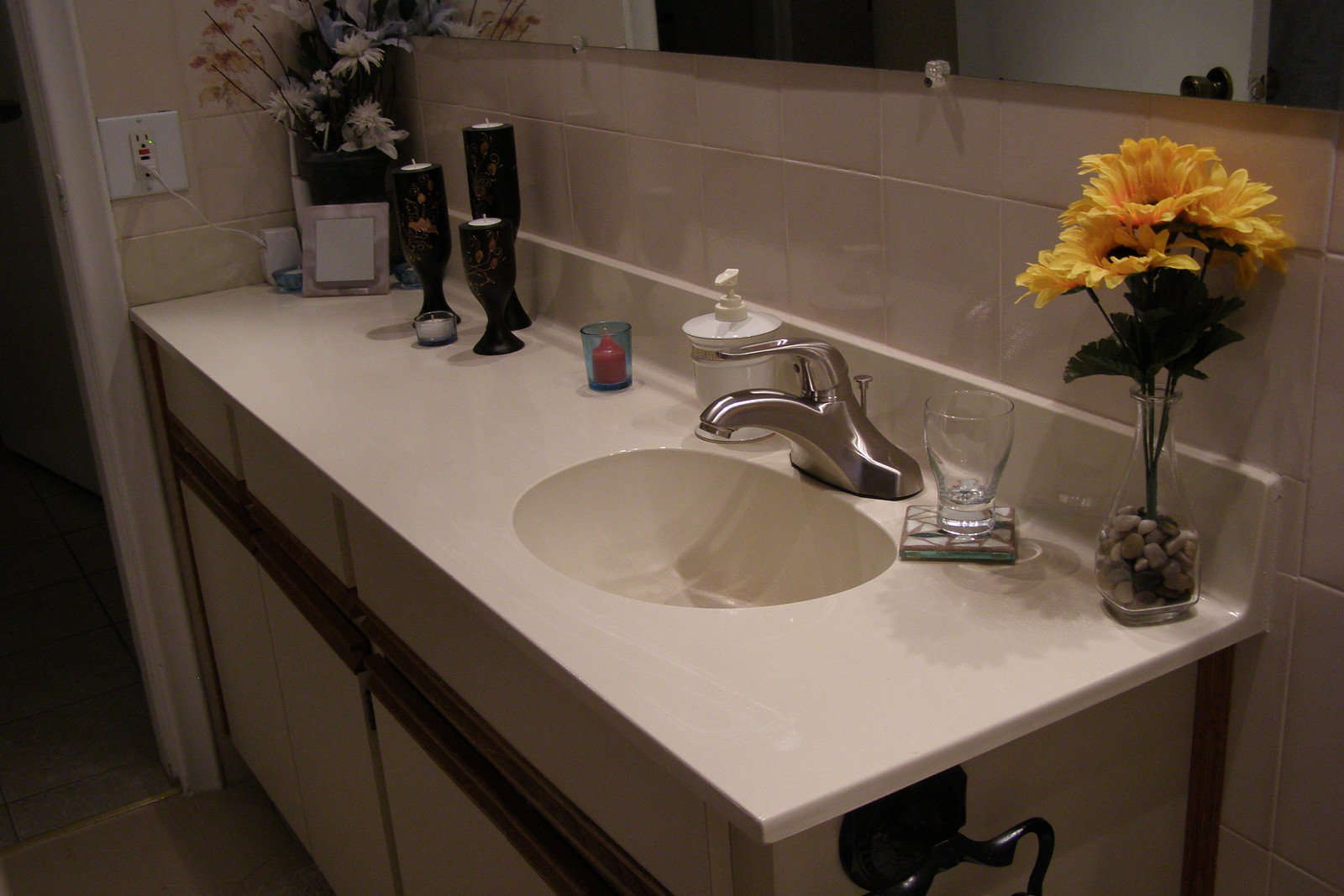The image captures the interior of a slightly older-style bathroom, indicative of a design from the late 1980s to early 1990s. The focus is on the countertop of the vanity which features integrated elements—a molded countertop with a built-in sink and backsplash. The silver faucet, traditional in appearance, adds to the dated aesthetic. To the left of the vanity, a doorway with white molding stands prominent against the wall, accompanied by a visible outlet plate.

The countertop displays a charming array of decorative and functional items. In the corner resides a bouquet of flowers, bringing a touch of freshness to the room. Nearby, three candle holders and a smaller standalone candle contribute to a cozy ambiance. Further right, a red candle encased in glass complements the scene. Practicality is evident with a pump soap dispenser placed to the left of the faucet, whereas a glass and an additional bouquet of flowers are situated to its right.

The bottom edge of a wall-mounted mirror peeks into the frame at the top, emphasizing the vanity area. Overall, the bathroom echoes a simple, yet nostalgic charm with touches of personal decor that hint at a bygone era.